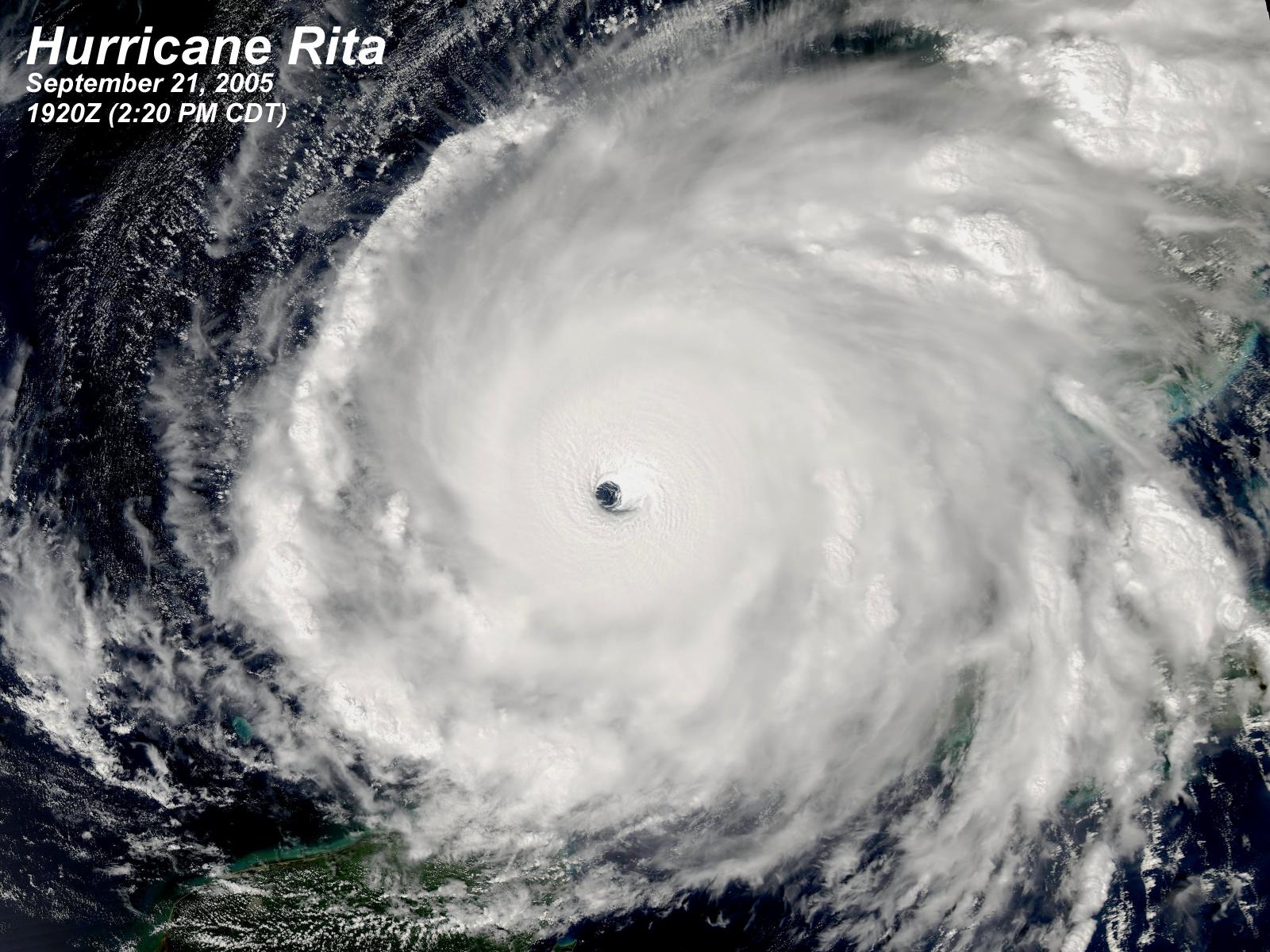This black and white aerial satellite image captures the powerful Hurricane Rita as it appeared on September 21st, 2005, at 1920Z (2:20 PM CDT). The text "Hurricane Rita" together with the date and time is clearly visible in white in the upper left corner of the image. Dominating the frame are the thick, swirling clouds of the hurricane, which form a massive spiral pattern over the dark, choppy waters of the ocean. At the very center of this spiral, the distinct eye of the storm—a near-perfect black circle devoid of clouds—stands out starkly. In the lower left and upper right corners, subtle patches of green indicate the presence of small landmasses or islands, adding a touch of color to the overwhelmingly monochromatic scene.